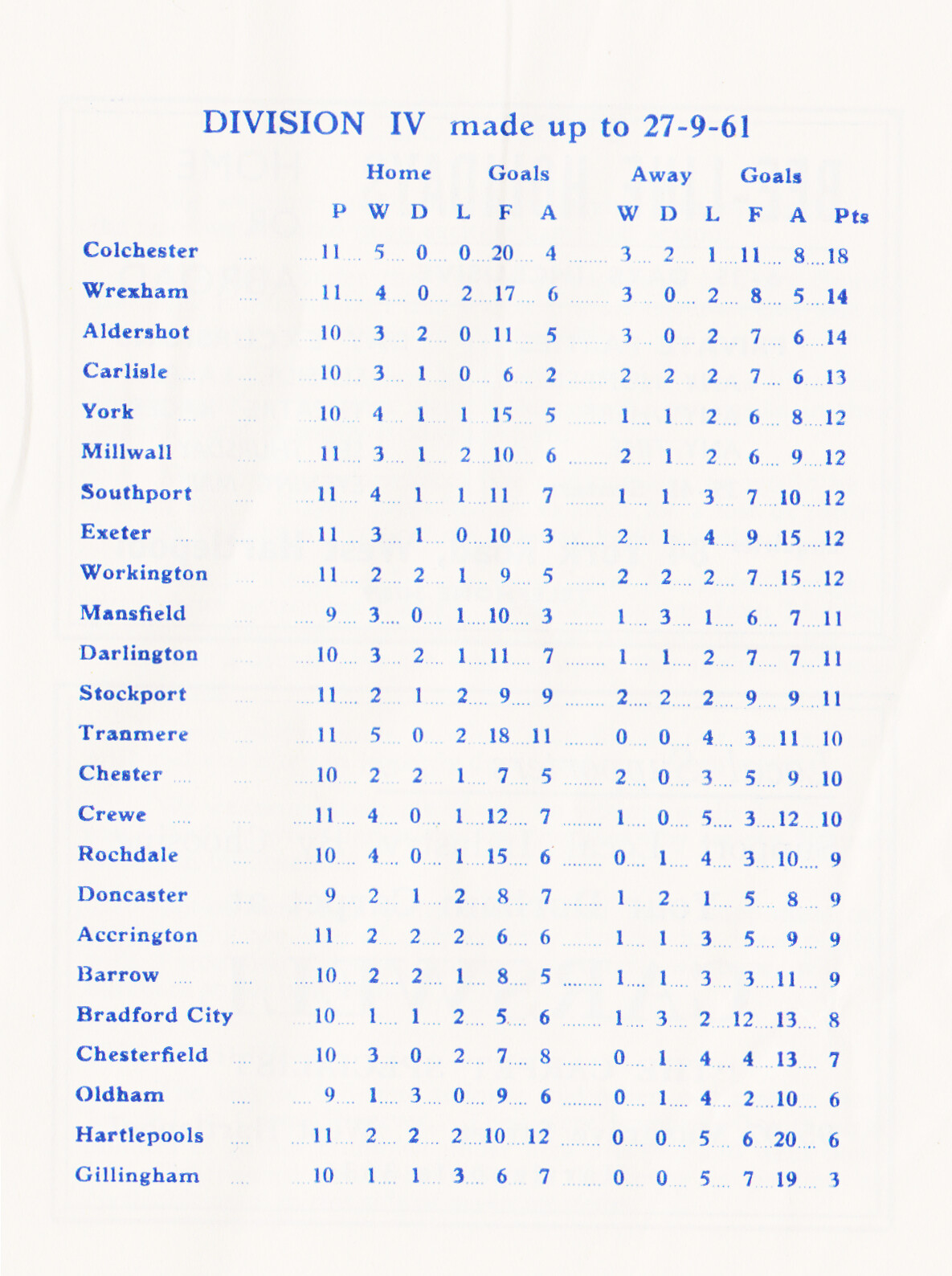The image features a white sheet of paper entirely filled with detailed sports information, likely from a scorebook or program related to Division 4 soccer teams, dated up to 27-9-61. At the top, written in blue, it prominently displays "Division 4, made up to 27-9-61." Below this, there are columns labeled "Home," "Goals," "Away," and "Goals" in blue text. Further down, abbreviations such as P, W, D, L, F, A under "Home" and corresponding W, D, L, F, A, and "Points" under "Away" categorize various match statistics. Team names, including Colchester, Wrexham, Aldershot, Carlisle, York, Millwall, Southport, Exeter, Workington, Mansfield, Darlington, Stockport, Tranmere, Chester, Crewe, Rochdale, Doncaster, Accrington, Barrow, Bradford City, Chesterfield, Oldham, Hartlepools, and Gillingham, are neatly listed down the left-hand side alongside corresponding numerical data. The sheet is predominantly blue and white, suggestive of a vintage sports document that might have appeared in a newspaper or sports magazine, and it presents the standings and statistics for the Division 4 soccer teams comprehensively.